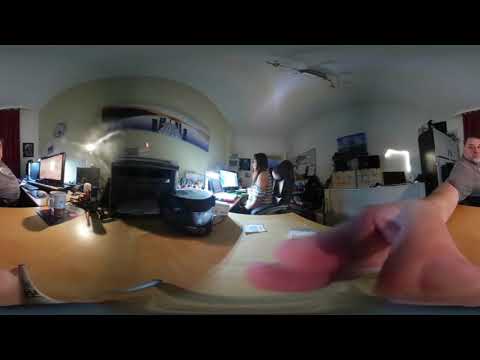The image is a 360-degree panoramic shot taken inside an office room with light green and white walls and a white ceiling. The photograph appears slightly blurred, framed horizontally with thick black borders at the top and bottom. It captures various people working at computers. 

In the center background, a young woman with long black hair, wearing a cold shoulder top with a striped pattern, sits on a black chair working at a computer. Directly in front of her is a large, brown rectangular desk on which a printer or similar device is placed. 

To the left, a heavyset man is partially visible, seemingly the same individual who is also on the right side of the picture. He is slightly cropped due to the panoramic effect, appearing distorted with a disproportionately small body and a large outstretched hand. His short sleeve gray shirt is noticeable as he reaches toward the camera, likely activating it, with his colossal finger evident in the bottom right-hand corner. The left side of the image reveals his midsection near another large monitor. 

Overall, the panoramic effect creates a surreal representation with each side of the image showcasing parts of the same person, many computers, and people engaged in their work within this detailed office setting.